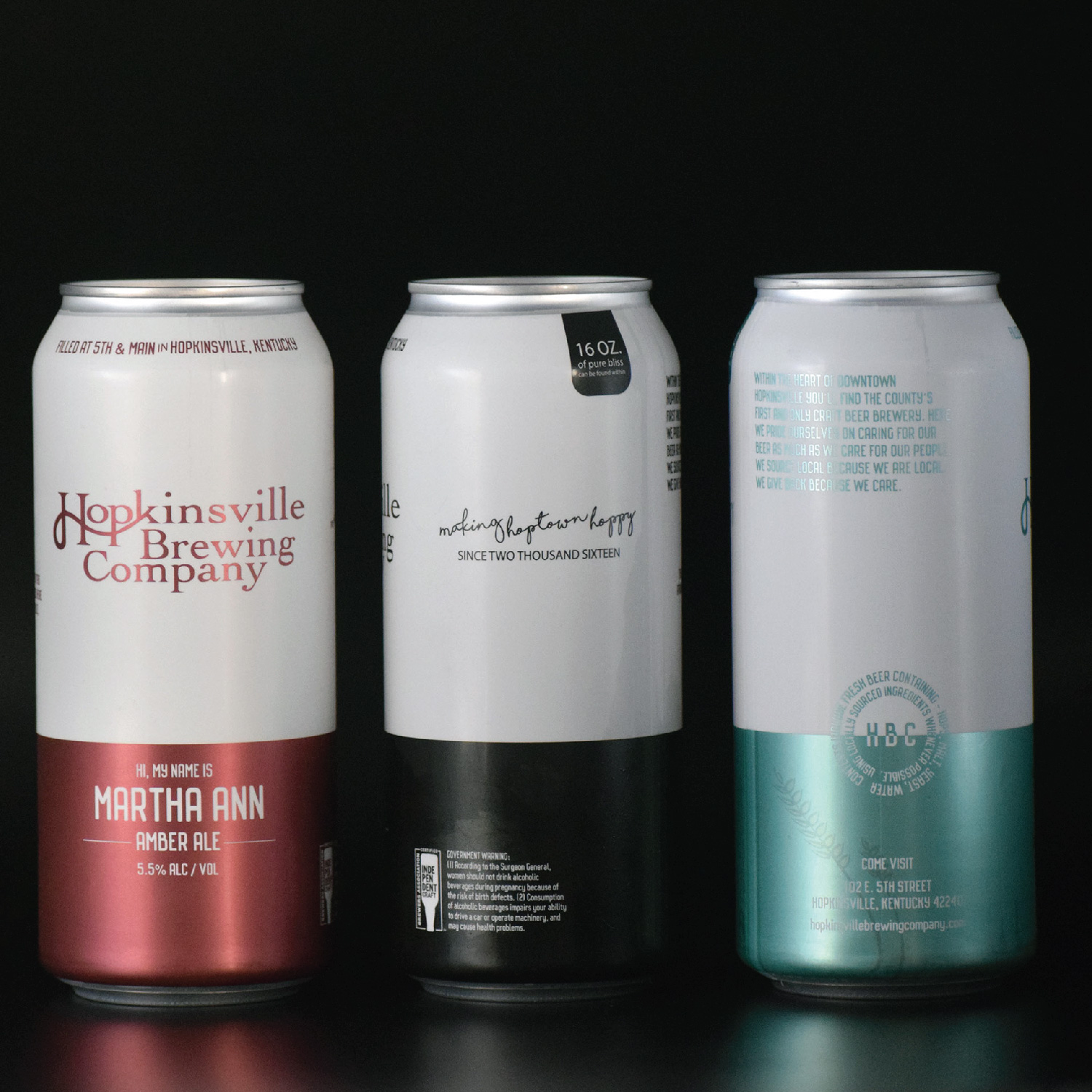The image features three cylindrical cans, each with a distinctive design, set against a sleek, black background and positioned on a highly reflective black surface. All the cans display a consistent design theme with the top two-thirds being white and the bottom third adorned with different colors. The can on the left has a rosy red bottom and reads "Hopkinsville Brewing Company" in red text in the white section, with additional text in white on the red section saying, "My name is Martha Ann, Amber Ale, 5.5% ALC per volume." The middle can features a black bottom and includes the phrase "Making Hoptown Happy Since 2016" in the white area and "16 ounces" near the bottom. The can on the right combines a white top with a light teal bottom, showcasing two circles of type and the abbreviation "HBC" at the transition from white to teal. The overall setup suggests a refined advertisement showcasing variations of beers from the Hopkinsville Brewing Company.